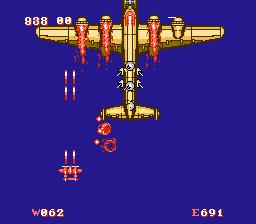This detailed screenshot from a pixel art-style video game features a dark blue background with a prominent top-view of a large, gold-colored bomber aircraft at the top. The bomber, depicted in pixel graphics, has four engines mounted on its wings, each trailing orange pixel flames, suggesting they are on fire or active. Despite the pixelated nature, the bomber displays shading with variations in gold tones.

To the left of the bomber is a smaller, red aircraft, possibly a seaplane, which appears to be launching an attack. It is shooting red-tipped rectangles, presumed to be missiles, towards the gold bomber. These projectiles have white centers and red extremities.

The bomber is equipped with small gray guns on its backside, indicated by circles and lines, totaling six – two on the left side, two on the right, and two on top. There are red explosions between the two planes, indicating active combat. 

Text elements on the image include a score of "9-3-8-0-0" in the top left corner, "0-6-2" in the bottom left, and "E 6-9-1" in the bottom right, likely representing player stats or game-specific data.